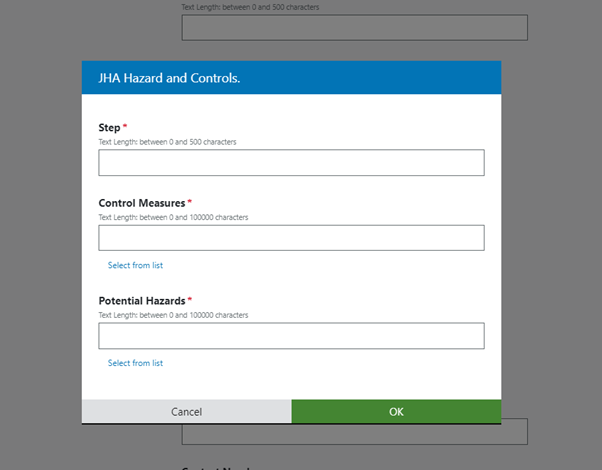**Caption:**

A screenshot of a settings menu from a web page, featuring a large, squarish pop-up box that covers most of the page. The background is gray, with the main pop-up window displaying a high-contrast blue band at the top, bearing the white text "J-H-I-A, Hazard and Controls." Below the blue band is a white section with detailed form fields.

At the top of the form, the heading "Step" is marked with a red asterisk, indicating a required field. This field has a specified text length limit between 0 and 500 characters, accompanied by a gray-outlined text box below it. Next, the section labeled "Control Measures," also marked with a red asterisk, allows for input lengths from 0 to 100,000 characters, with an associated text box.

Within the white section, "Select from list" appears in blue text underneath both "Control Measures" and "Potential Hazards" sections. The "Potential Hazards" section, again marked with a red asterisk, specifies a text length limit of up to 100,000 characters, similar to "Control Measures."

At the bottom of the pop-up window, on the left side, there’s a gray "Cancel" button with black text and a green "OK" button with white text. A thin black band runs along the bottom of the pop-up window, completing the interface.